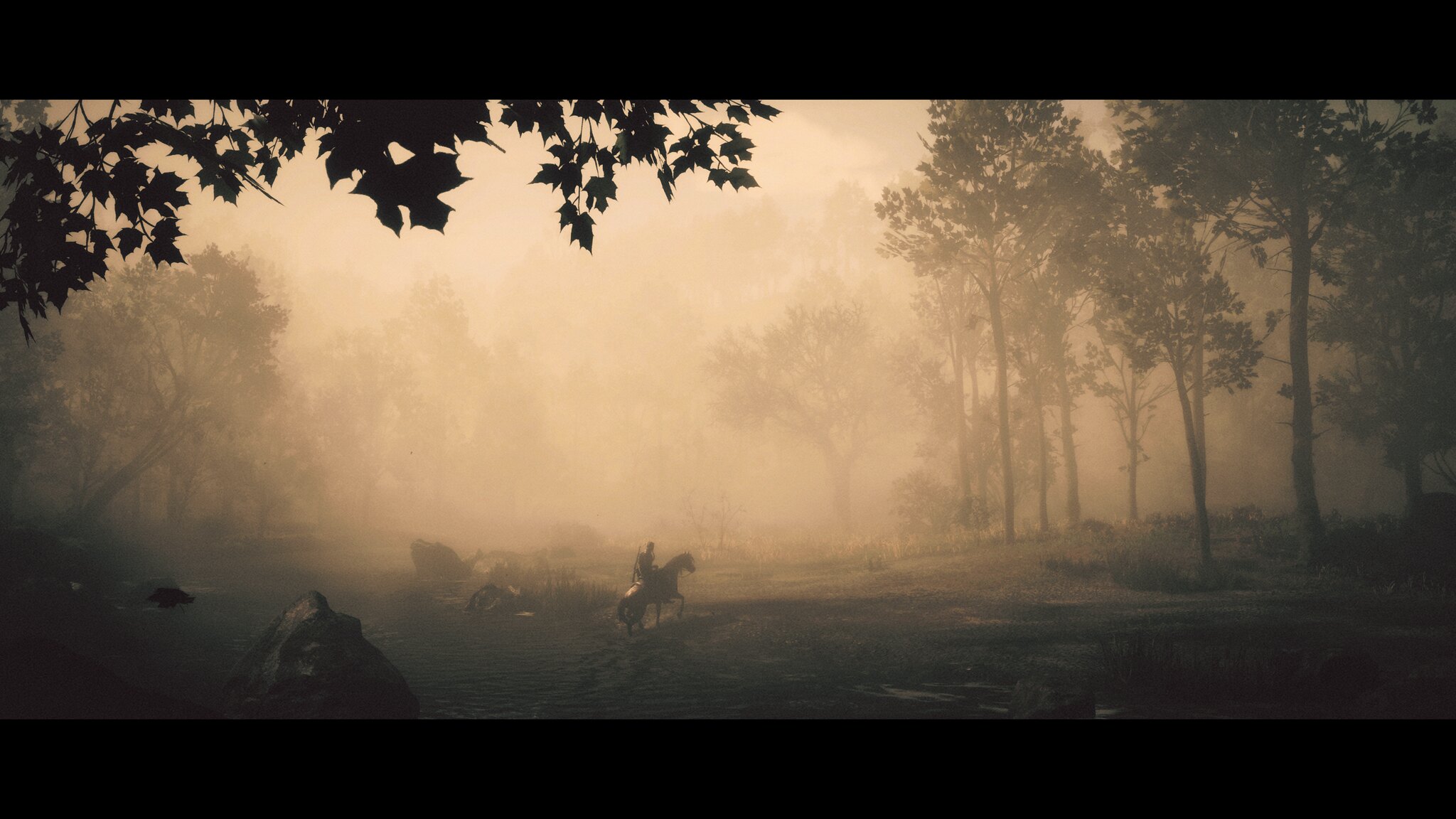A sepia-toned photograph-style image depicts a haunting battlefield scene. Framed by black bars at the top and bottom, the image is imbued with a somber atmosphere. At the top, a leafy branch is partially visible, adding a touch of nature to the otherwise grim setting. The ground below is wet and muddy, with puddles scattered across the field. In the center, a horse stands amidst the muck, ridden by a lone figure. In the foreground, a person is seen crawling through the dirt, their struggle palpable. Surrounding the scene are trees with varying amounts of foliage, creating a backdrop that ranges from sparse to dense. In the background, several fallen figures can be seen, adding to the sense of despair. Sunlight pierces through the scene, casting an eerie light that highlights the somber mood of the battlefield.